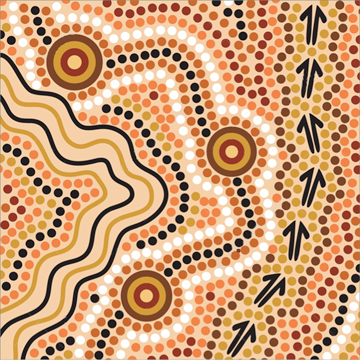This abstract digital drawing displays a complex and detailed arrangement of various shapes and colors on a light peach background. The composition includes curving patterns formed by rows of solid-colored beads in black, orange, green, white, and gold, spaced perfectly apart, creating a grid-like appearance across the entire artwork. Prominent within the piece are three large circles, each consisting of layered colors: brown, light brown, red, and beige. Additionally, there is a recurring motif of black squiggly lines interspersed with gold lines, resembling bacon stripes. These lines enclose smaller circular patterns featuring colors like orange, black, gold, and peach. Among the elements, a distinctive group of seven black arrow-like shapes moves upward in a sequence, resembling Pac-Man figures—these arrows appear to be interacting with the surrounding beads. The intricate and layered details combine to form a vivid and dynamic piece of graphic art.